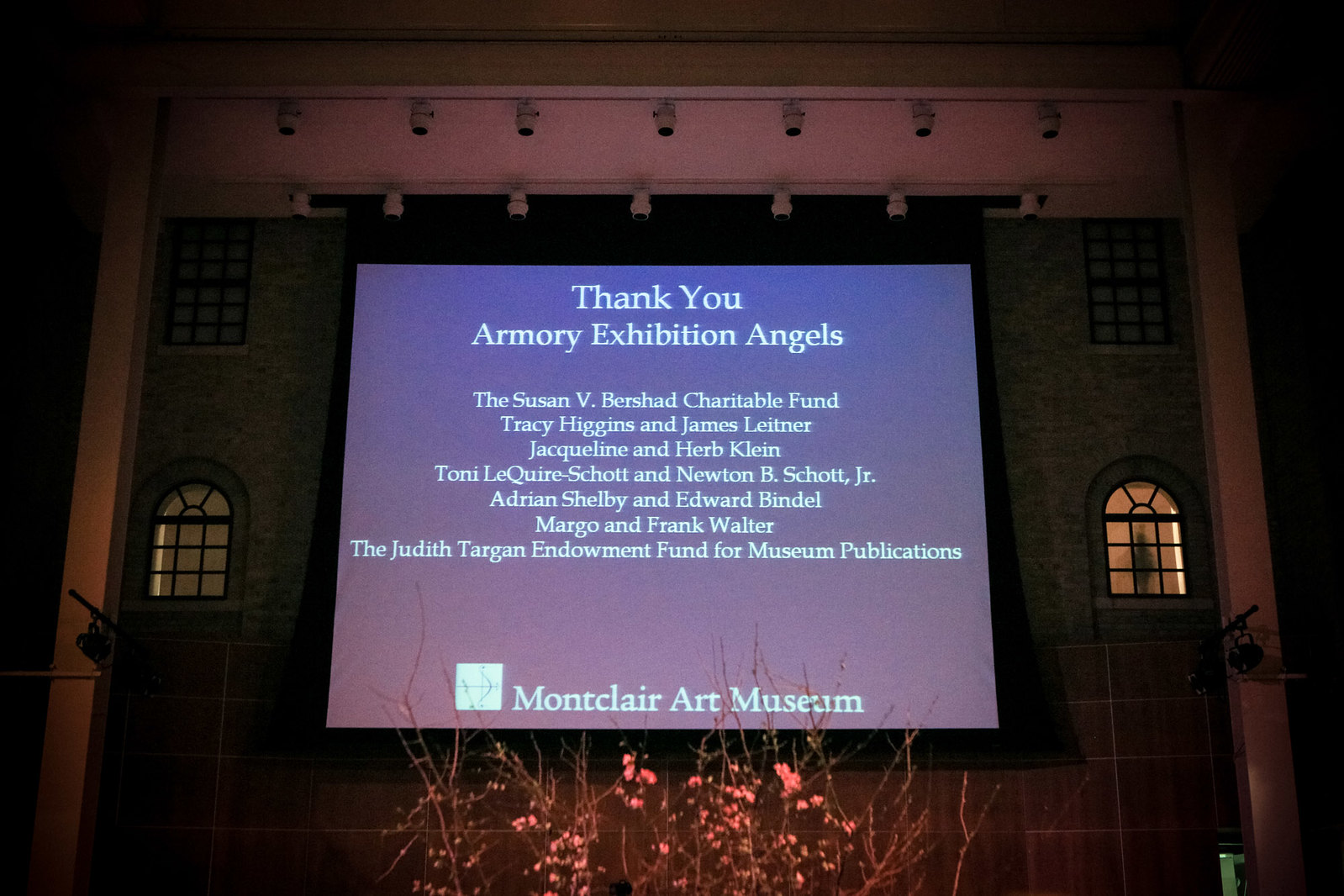The image depicts a photograph of a staged setup resembling the exterior of a building, with a large projection screen mounted on the wall. The screen has a gradient background of blue and pink, with white text that reads, "Thank you, Armory Exhibition Angels, the Susan B. Bershaw Charitable Fund, Tracy Higgins and James Leitner, Jacqueline and Herb Klein, Tony Lequaire Scott and Newton B. Scott Jr., Adrian Shelby and Edward Bindel, Margot and Frank Walter, the Judith Targon Endowment Fund for Museum Publications." At the bottom of the screen, the text reads "Montclair Art Museum." The setup includes stage lighting above the projection screen and a total of 14 lights. On either side of the screen, the building façade features two windows on the left and two on the right; the lower ones are arched with glass doors, while the upper ones are rectangular. Visible at the bottom are dried shrubs with pink flowers. Additionally, above the screen, there are numerous framed pictures arranged in a line, enhancing the appearance of the setting.